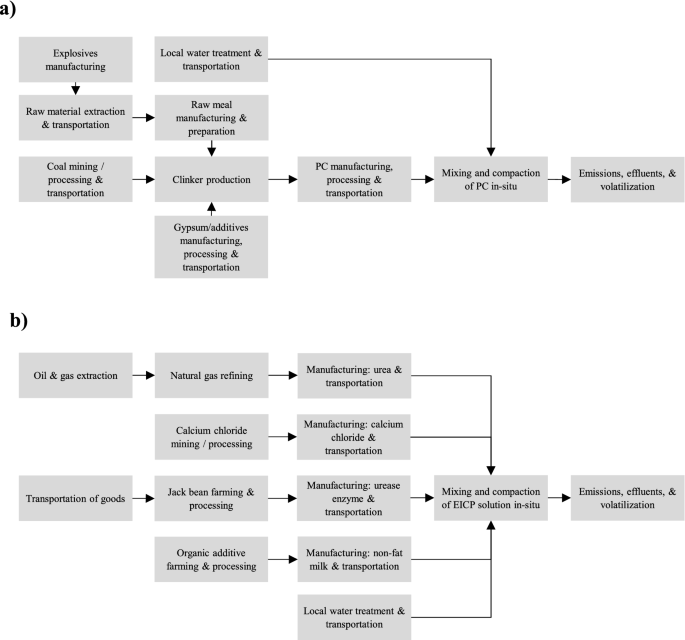The image displays two detailed workflow diagrams labeled 'A' and 'B,' highlighting extensive manufacturing processes. In Diagram A, the sequence begins with 'Explosive Manufacturing,' moving downward to 'Raw Material Extraction and Transportation,' followed by a horizontal shift to the right toward 'Coal Mining, Processing, and Transportation.' From there, it proceeds downward to 'Clinker Production' and rightward to 'PC Manufacturing, Processing, and Transportation.' Additional stages include the 'Mixing and Compaction of PC in Stu' and culminates in 'Emissions, Effluents, and Volatilization.'

Diagram B begins at the top left with 'Oil and Gas Extraction,' followed by a rightward arrow to 'Natural Gas Refining.' The process continues to the right with 'Manufacturing of Urea and Transportation,' involving additional complex stages like 'Mixing and Compaction of EICP Solution in City,' and concludes with 'Emissions Influence and Volatilization.' Both diagrams illustrate interconnected steps involving resource extraction, processing, and final product manufacturing, emphasizing environmental impacts through emissions and effluents in the final stages.